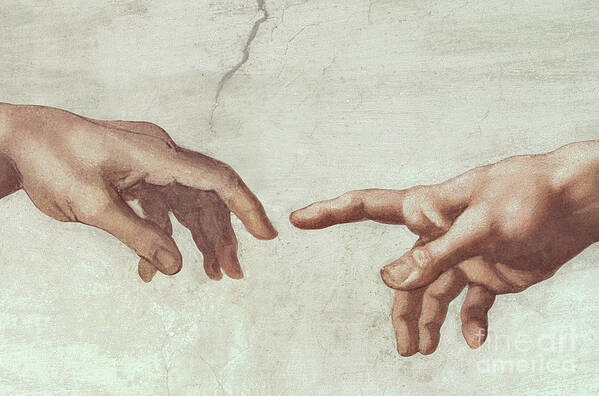This image is a detailed section of Michelangelo's famous artwork, *The Creation of Man*, specifically focusing on the two hands reaching towards each other. Both hands, rendered in shades of pale white, light cream, and beige, are open with fingers extended, creating a moment of almost-touching index fingers. The left hand, coming from a higher position, points diagonally downward, while the right hand, emerging slightly lower, mirrors this with its finger angled upward. Only the hands from the wrists forward are visible. The backdrop is a textured, grayish-green and light cream surface with visible cracks, notably a prominent crack descending from the top above the left hand. A faint watermark reading "fine art america" is present in the bottom right corner, blending subtly into the background.